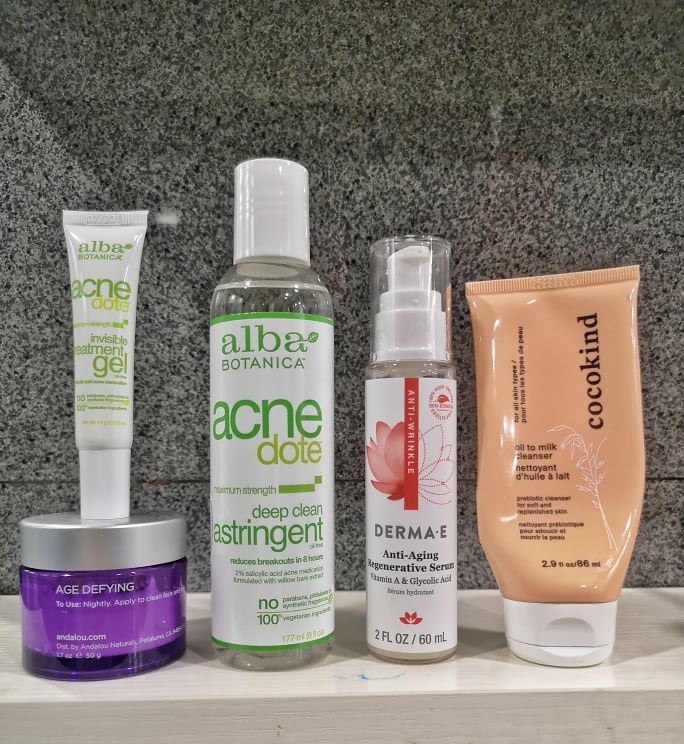In the image, several skincare products are meticulously arranged in a row on a countertop against a marbled gray wall. On the far left sits an age-defying cream in a purple jar, with a small acne gel product perched on top of it. To its right, there is a clear plastic bottle featuring a green and white label of Alba Botanica's 'Acne Dote Astringent.' Following this, a smaller plastic bottle containing Derma E's Regenerative Serum, an anti-wrinkle product, is positioned. Finally, on the far right, there is an oil-to-milk cleanser by the brand Coco Kind. All the products are ordered from left to right. Additionally, situated at the lower center of the image in front of the Derma E serum, there is a noticeable blue smudge on the countertop. The overall arrangement displays a visually appealing and organized presentation of various skincare essentials.